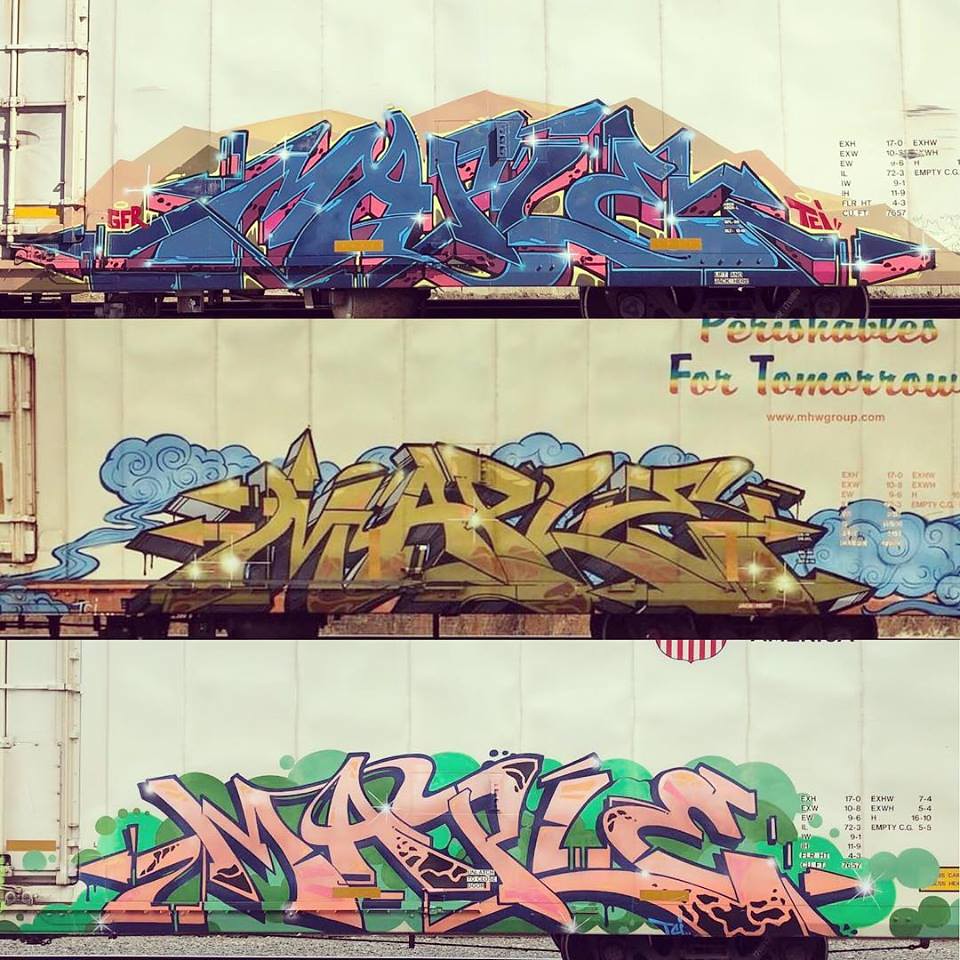The image is slightly taller than it is wide and is divided into three horizontal sections, each showcasing different graffiti designs with a shared light yellow background segmented by light brown vertical lines into around ten sections each. 

In the top section, the backdrop features a range of five interlocking mountain peaks in varying shades of brown and red-brown. Overlaid on this rugged terrain are 3D blue letters edged with pink, some of which sparkle at the corners. Prominent letters include M and A.

The middle section presents a background of serene blue clouds. Superimposed on this are 3D yellow letters, with a notable inscription reading "perishables for tomorrow" at the top right. The letters exhibit some rainbow-like coloration, and letters such as M, A, and P are discernible.

In the bottom section, a green, smoky, and somewhat bubbly background sets the scene for 3D bubble letters in a light pink hue. The graffiti appears on what might be a metal silo, completing a vibrant and varied street art display that merges natural elements with urban creativity.